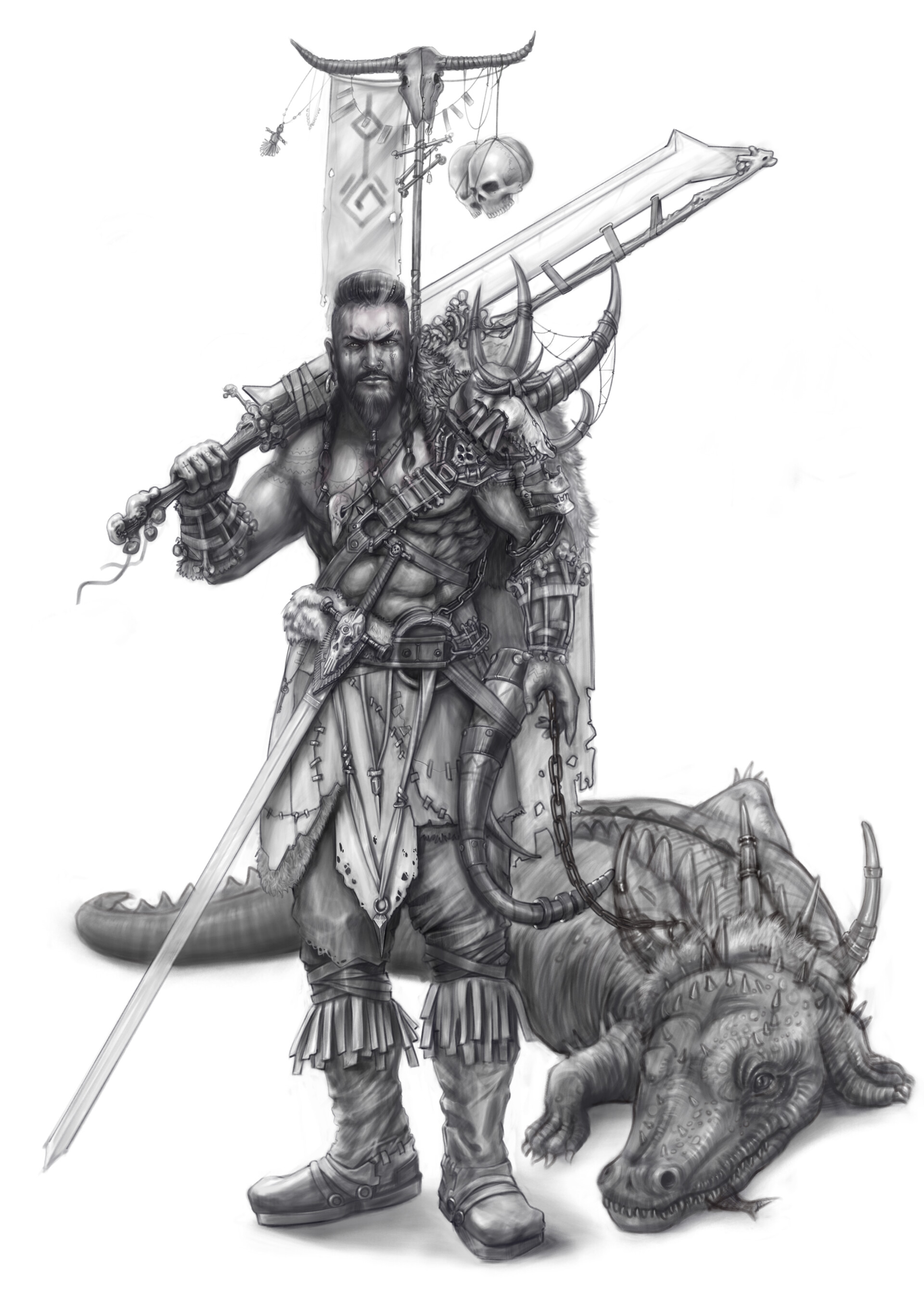This highly detailed pencil drawing, set against a stark white background, depicts a muscular warrior, outfitted with an array of weapons and accessories. The warrior, clad in a costume featuring knee-high boots that are strapped at the top and a skirt made of animal skin, exudes a fierce and rugged presence. His eyes are braided, and he sports various piercings, enhancing his intimidating look. He holds a large, handmade blade with what appear to be antler-like features. Strapped to his back are additional weapons, including something that resembles a saw. At his side, tethered to a chain, is a formidable crocodile, its mouth clamped around a fish, with the fish’s tail protruding. Above the warrior hangs a collection of macabre items, including animal skeletons, human skulls, and a flag, further accentuating the image's raw and primitive atmosphere.